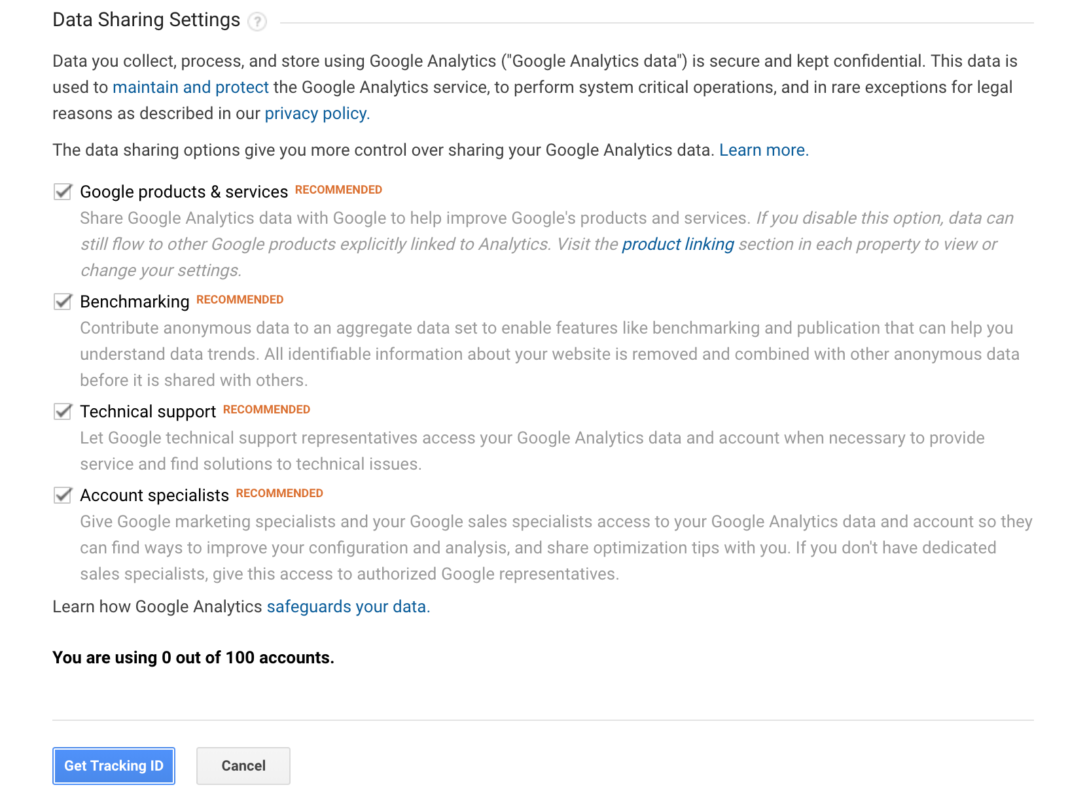**Caption:**

This image captures the data sharing settings section of the Google Analytics interface. The section details how data collected, processed, and stored using Google Analytics is handled. It emphasizes that this data is secure and kept confidential, being utilized to maintain and protect the Google Analytics service, perform system-critical operations, and, in rare cases, for legal reasons as specified in Google's privacy policy.

The settings also highlight the data sharing options available to users, providing more control over their Google Analytics data. 

Below this description, there are four options, each accompanied by a checkbox that has been checked:

1. Google products and services
2. Benchmarking
3. Technical support
4. Account specialists

Additionally, there is a note that users can learn more about how Google Analytics safeguards their data.